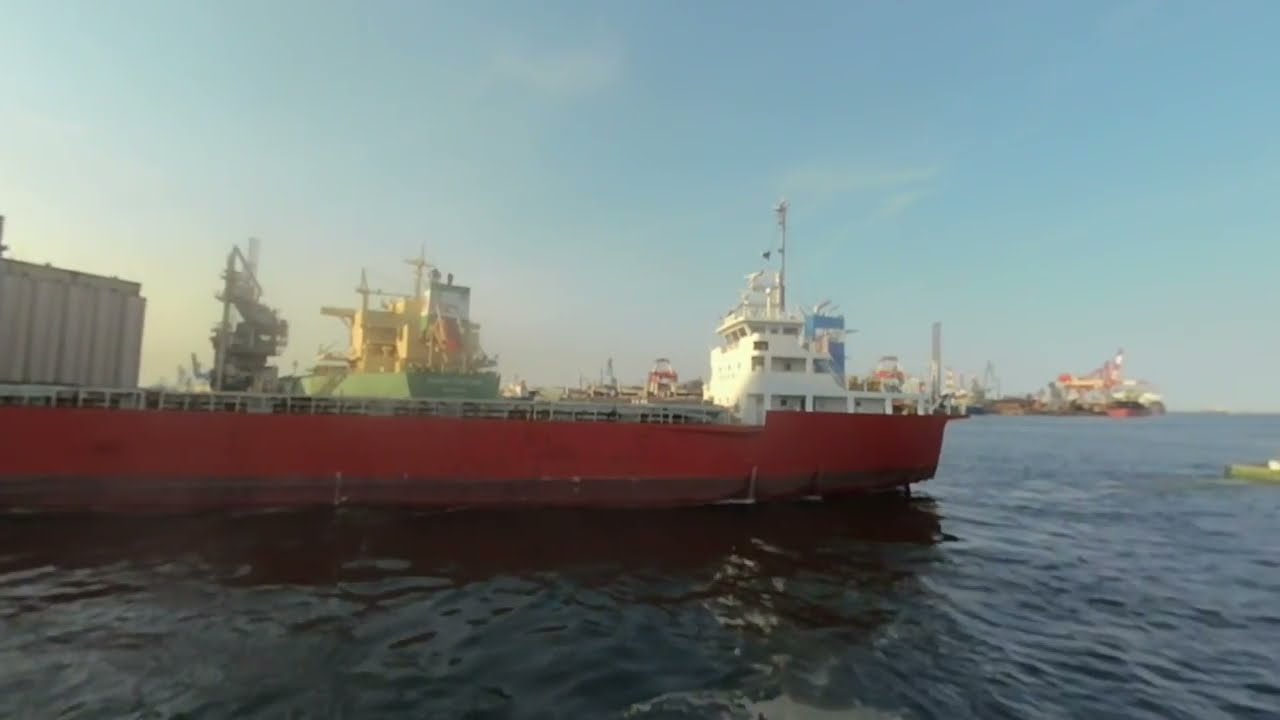In the image, there is a massive red cargo ship floating on calm, dark blue water, potentially in a shipyard or loading facility. The vessel is predominantly red, extending from the left-hand side almost to the far right of the image, with a notably flat and bare deck that appears devoid of cargo. The front part of the ship features a tall white superstructure, replete with balconies, doorways, windows, and various antennas on top. Just to the left of the red vessel, there is another distinct vessel colored green and yellow, while to the far right in the distance, another vessel emerges, possibly an oil rig or a crane-equipped structure. Additionally, a gray container is visible on the deck of the red ship. The backdrop is a clear sky with hardly any clouds, enhancing the bright, sunlit atmosphere. The scene suggests a bustling shipping area, with large cranes and other vessels in the background, emphasizing the industrial surroundings. There are no people visible in the entire photograph.